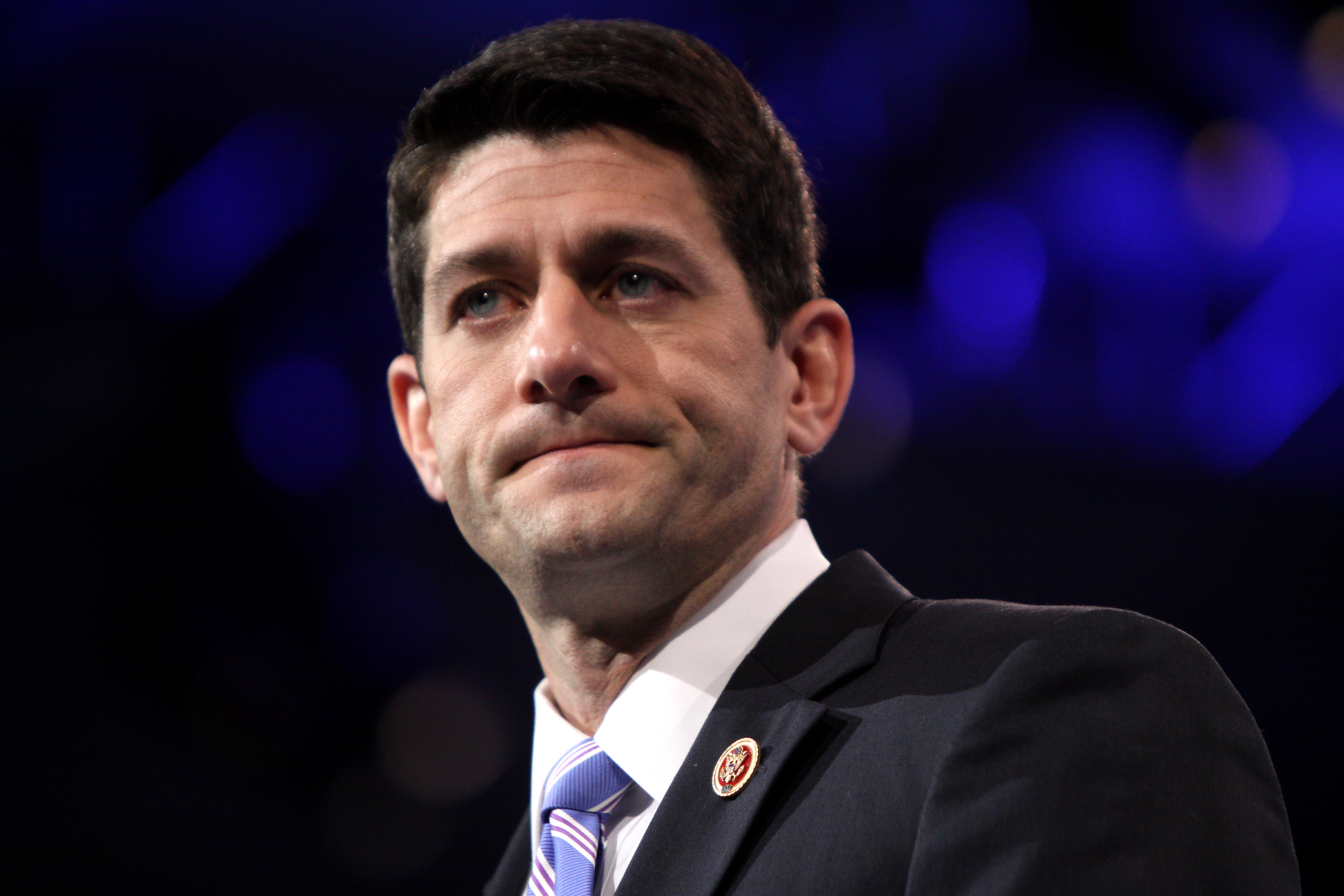This image features Paul Ryan, the former Speaker of the House, at the very center with the backdrop dramatically blurred. The photograph captures Ryan from just below the shoulders upward as he looks intently off to the left, his expression appearing concerned or perhaps disappointed, with his lips pursed and dimples visible. He has light skin, blue eyes, and very dark brown to black short hair. He is dressed in a black blazer adorned with a small circular gold and red pin featuring an eagle insignia. Underneath, he wears a white collared shirt paired with a light blue necktie striped with red and white. The background is primarily black, transitioning to blue and possibly shades of purple, with the lights creating a bubble-like effect that adds a dramatic contrast to his formal attire.